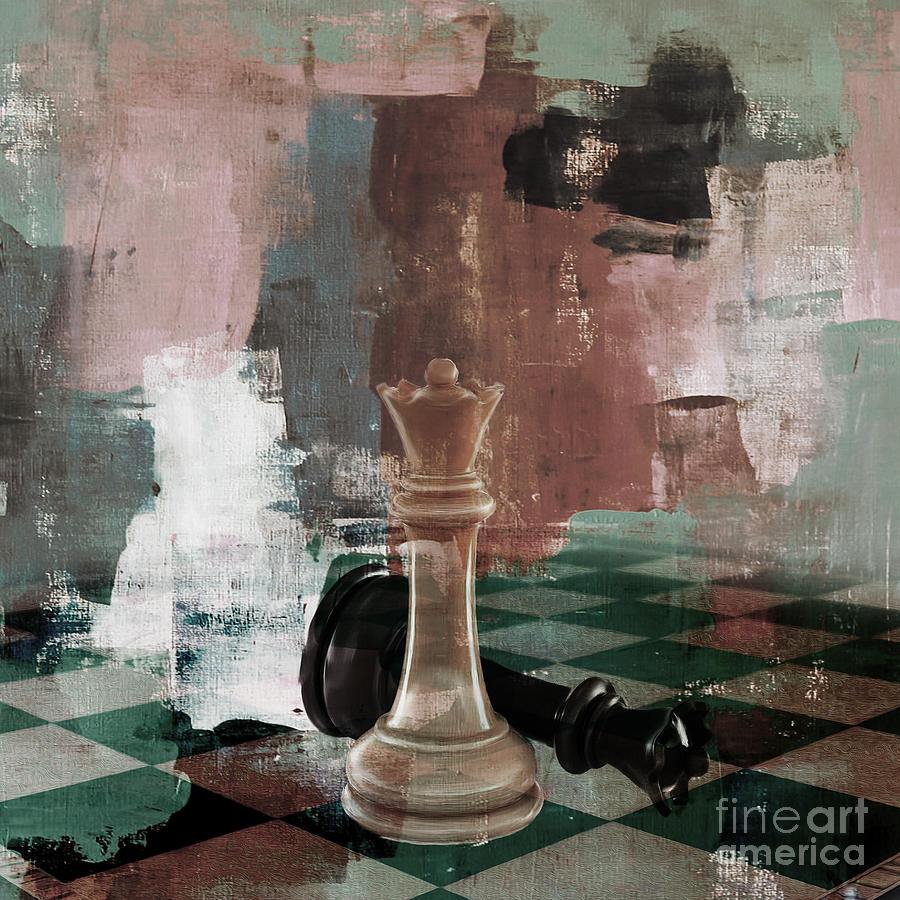This is a square abstract painting featuring a chessboard in the foreground with a light gray and black checkered design. Dominating the scene is a standing, brownish-white Queen chess piece. Directly behind and partially obscured by this white Queen is a toppled black Queen piece, with its base visible on both sides of the white Queen. The background is a vibrant explosion of colors with smeared and splotched reds, whites, greens, blacks, and hints of pink, light blue, and teal. Despite the predominance of abstract brushstrokes and color swipes, the chessboard and pieces remain the focal point. The painting bears a light gray watermark in the bottom right-hand corner that reads “Fine Art America.”